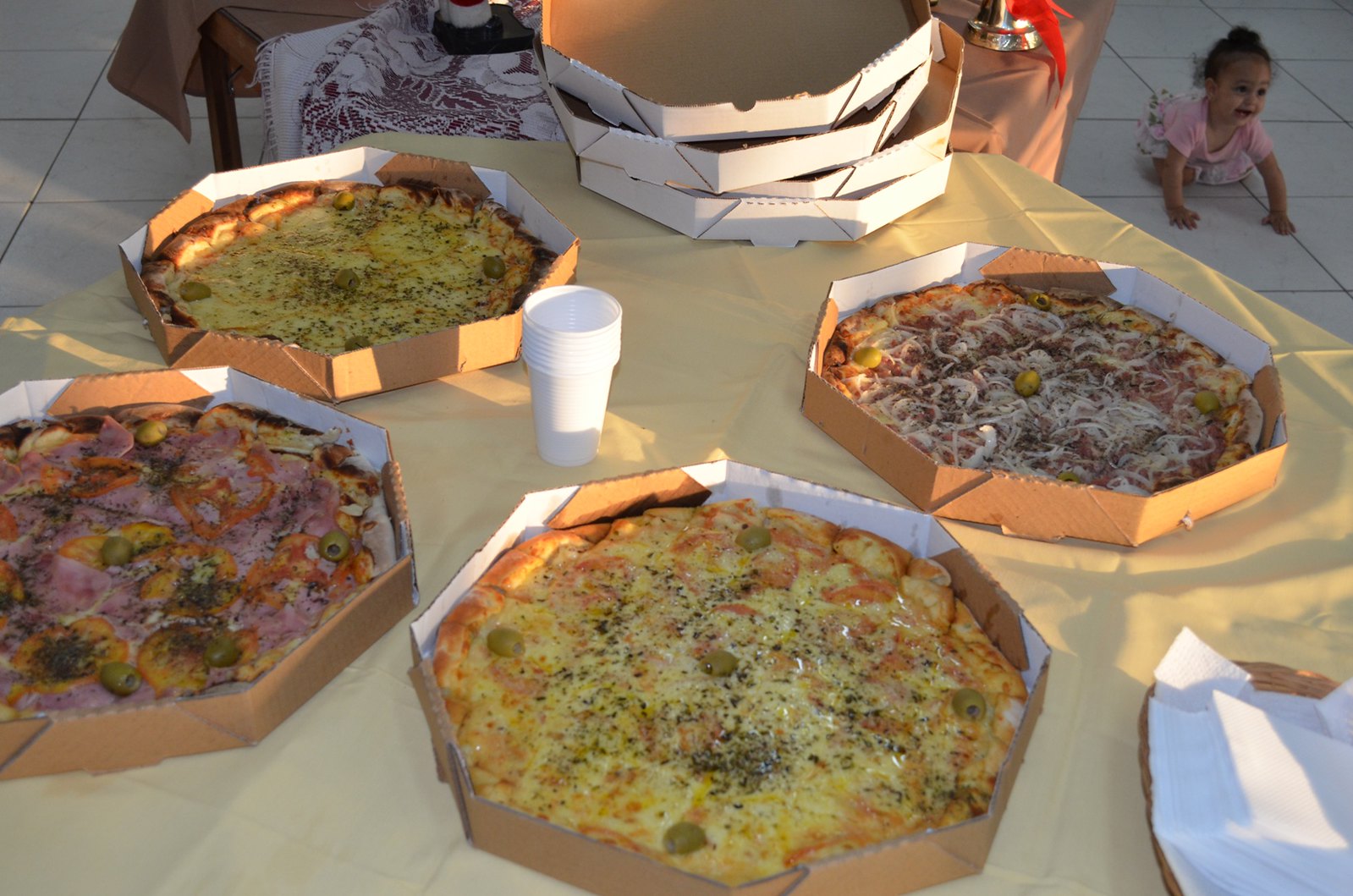In an image of a table with a yellow plastic tablecloth and white tiled floor, there are four small, individually topped, octagonal pizzas placed in brown cardboard boxes with white interiors. Each pizza sports different toppings: one appears to have just cheese, another includes cheese and olives, a third features a mix of meats, red peppers and possibly tomatoes, and the fourth showcases a different variety of cheese with more olives. In the center of the table, there's a stack of white Styrofoam cups, and at the top of the image, the lids to the pizza boxes are visible. On the floor nearby, a toddler girl with frizzy dark hair is seen wearing a pink shirt and white ruffled bottoms. A second table is visible behind the pizza table.